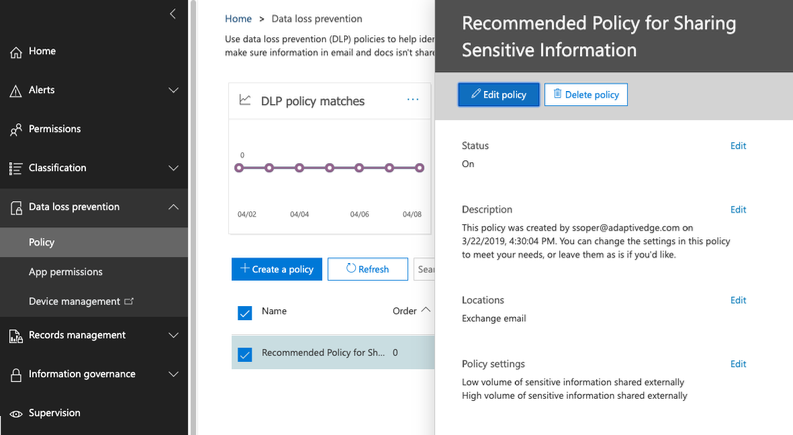This image captures a detailed administrative interface, displaying various options and configurations related to data management and security. The screen presents several tabs, including "Home," "Alerts," "Permissions," "Classification," "Data Loss Prevention," "Policy," "App Permissions," "Device Management," "Records Management," "Information Governance," and "Supervision." The central part of the image focuses on the "Data Loss Prevention" (DLP) section, highlighting tools and guidelines for preventing unauthorized sharing of sensitive information through emails and documents. It also features a policy, labeled "Recommended Policy for Sharing Sensitive Information," which was created by S Supa from adaptiveedge.com on March 22, 2019, at 4:30 PM. The interface allows users to edit or delete this policy, and provides a status description. Users are given the option to customize the policy settings to fit specific needs, or to retain the default configurations.